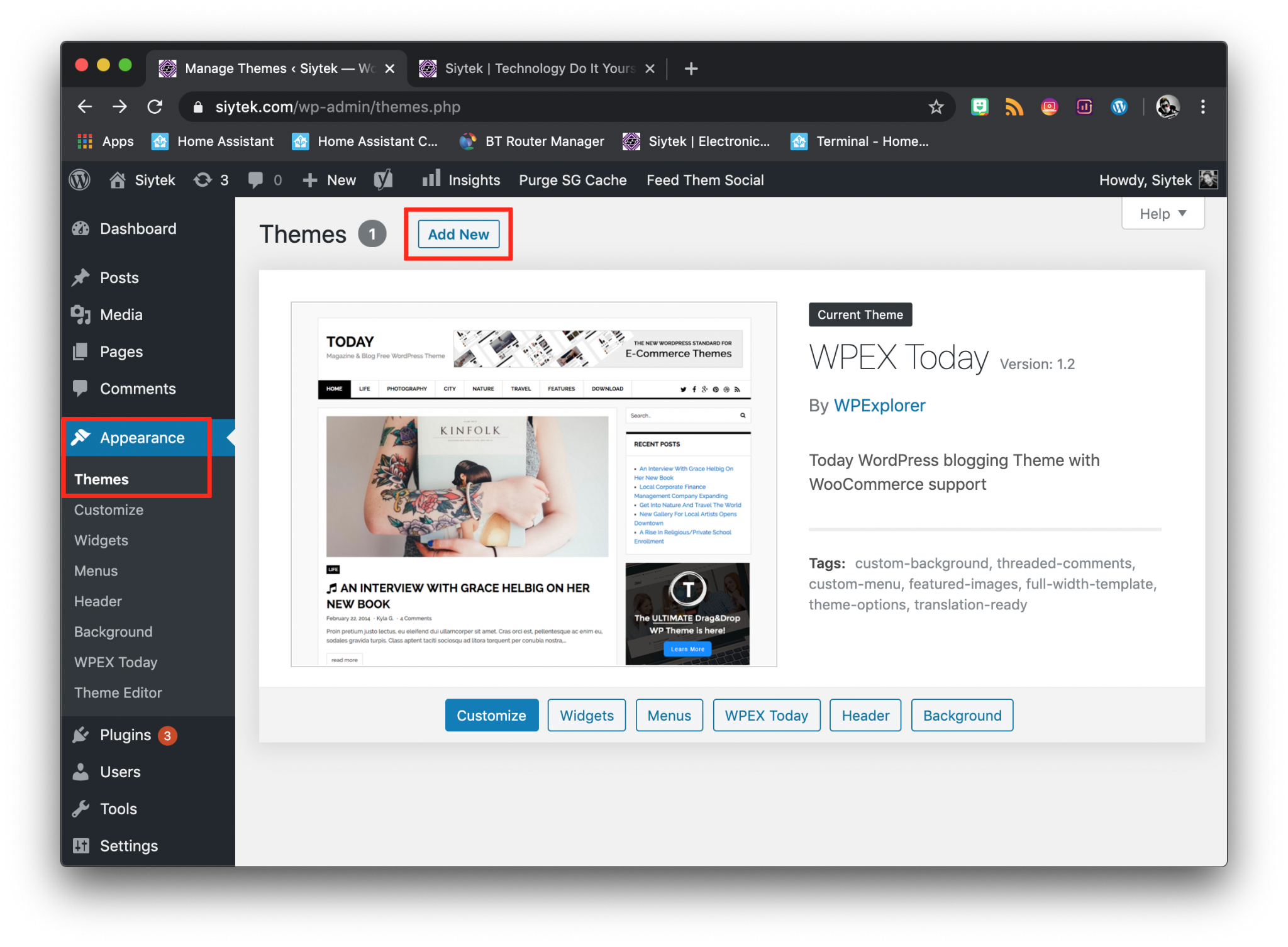**Detailed Caption:**

The screenshot showcases a web browser with the dark mode enabled, displaying two open tabs at the top. The active tab is titled "Managed Themes" on the administrative dashboard of siytekscitech.com, specifically at the URL wp-admin/themes.php. The secondary tab, although open, remains inactive and is labeled "SciTech Technology DIY."

Below the search bar, the browser features several quick access bookmarks, including "Apps," "Home Assistant," "BT Router Manager," "SciTech," and "Terminal." The visible webpage is a WordPress dashboard, identifiable by the WordPress icon in the top left corner and various menu items.

The sidebar menu indicates the user is working on the "Appearance" section, highlighted in blue with a white paintbrush icon. The central content area displays the "Themes" screen, with the "Add New" option also highlighted in blue against a gray background.

The primary theme shown here is "WPEX Today" version 1.2, described as a "WordPress blogging theme with WooCommerce support." The theme visual preview demonstrates a clean, newspaper-like layout featuring an interview with Grace Helbig about her new book, structured in a blocky, vertical format with white, gray, and black elements.

Listed tags for the theme include "Custom Background," "Threaded Comments," "Custom Menu," "Featured Images," "Full Width Template," "Theme Options," and "Translation Ready." Users can further manage the theme using buttons beneath the preview, such as "Customize," "Widgets," "Menus," "WPEX Today," "Header," and "Background," each marked with blue text and rectangles.

The WordPress dashboard’s left-hand menu extends to additional functionalities like "Plugins," "Users," "Tools," and "Settings," offering comprehensive site management options.